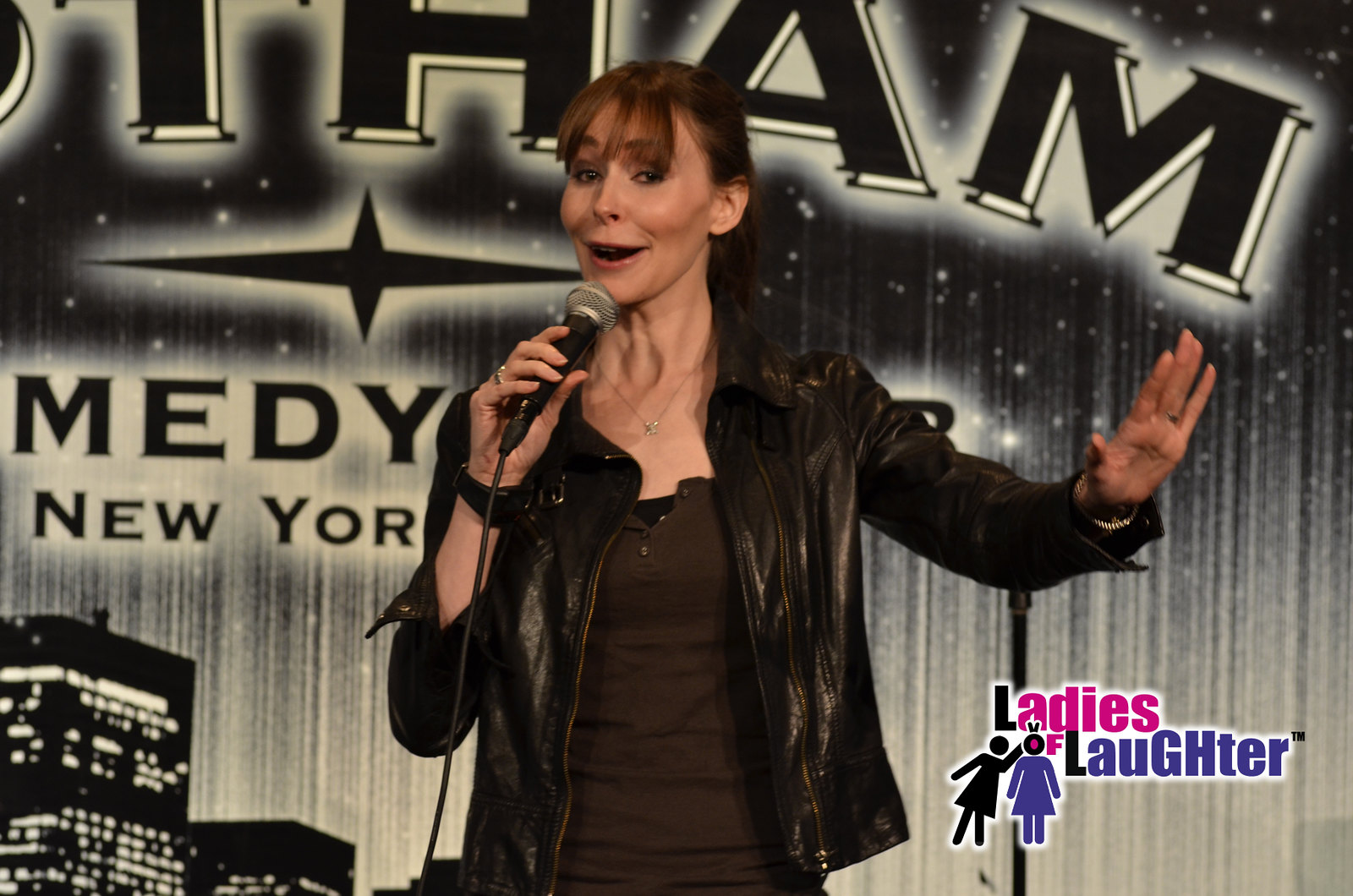In this detailed photograph, a mid-aged, pale-skinned woman with brown-red, shoulder-length hair stands on stage performing a comedy routine. She is dressed in a black faux leather jacket over a brown blouse and accessorized with a watch on her right wrist and a ring on her finger. She holds a microphone in her right hand, which is extended, as her other hand gestures outward. The backdrop features a dark, star-studded pattern with building silhouettes and a partially visible logo that reads "Gotham Comedy Tour" indicating the New York club setting. Prominently placed in the bottom right corner is a vibrant logo in pink, purple, and blue colors, captioned "Ladies of Laughter," accompanied by emoji-like female figures. The backdrop is a mix of green and black hues, enhancing the playful yet professional atmosphere of the comedy event.